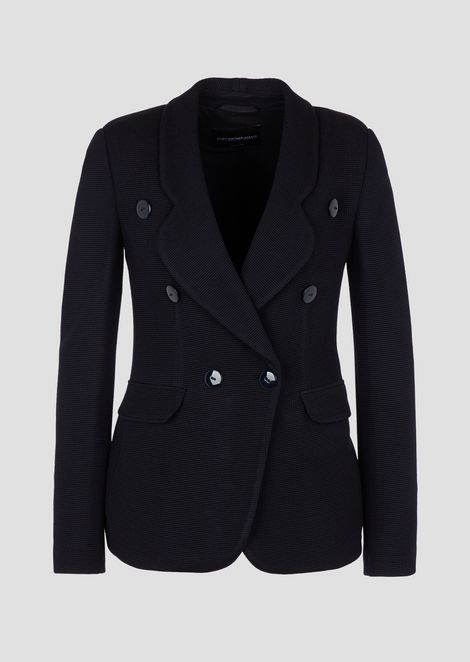The image depicts an elegant black designer coat, meticulously centered against a plain gray background. This sophisticated button-down coat lacks a zipper and features six prominent buttons, three on each side. The coat, directly facing the camera, gives off an air of high fashion, reminiscent of luxury clothing suitable for a high-end retailer. It boasts wide lapels and two pockets situated near the hips. Despite its formal appeal, the coat is not displayed on a mannequin, instead appearing to be effortlessly hanging in mid-air. The refined craftsmanship and detailed elements, such as the long, narrow sleeves and the reflective accents of white from the lighting, suggest it's an expensive, possibly women's garment you might find in an upscale boutique.